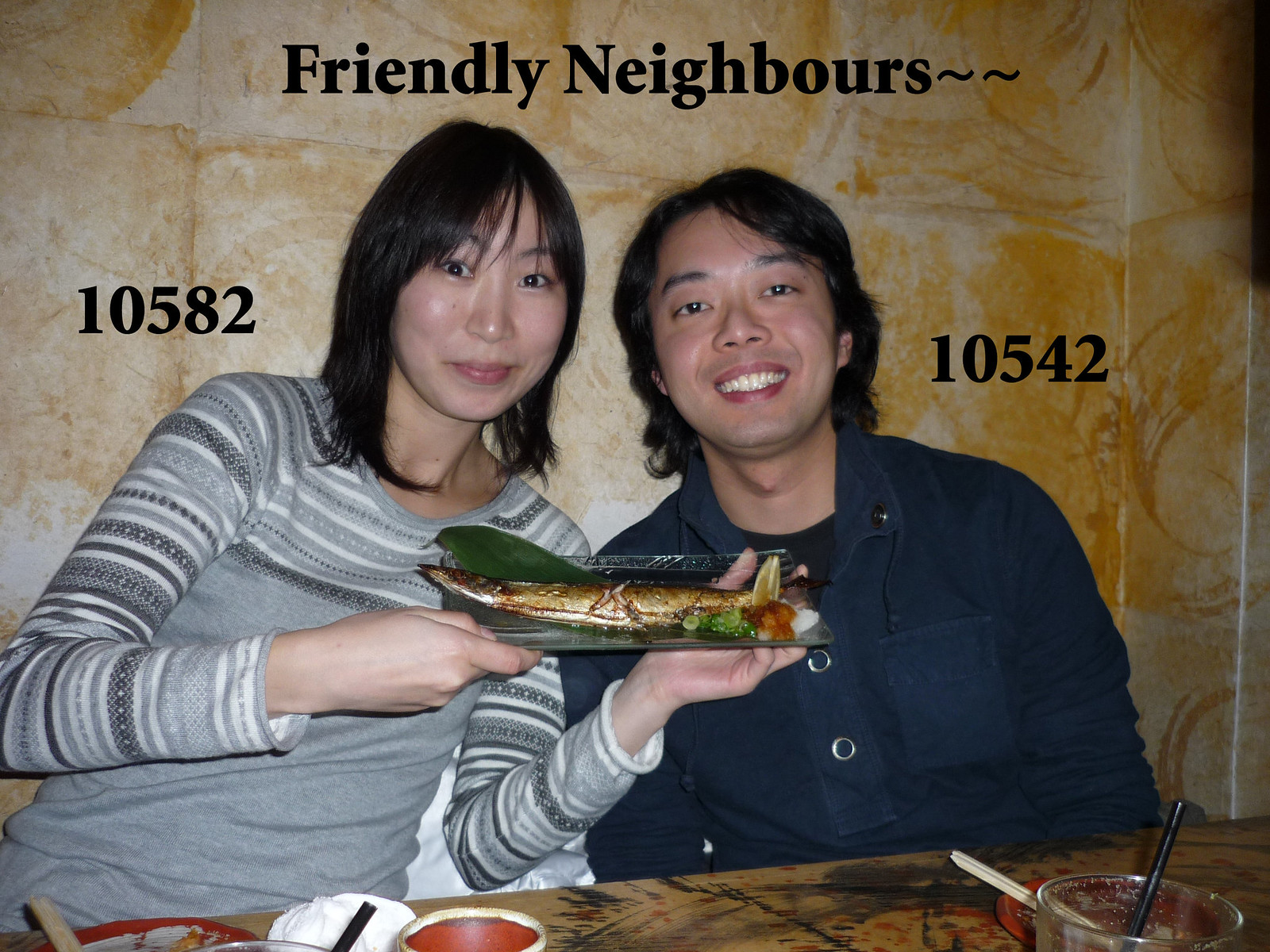In this warm and vibrant photograph, two smiling Asian individuals are seated at a restaurant table, posing cheerfully for the camera. The woman on the left, who has shoulder-length black hair, is dressed in a gray sweater adorned with colorful stripes on the top and sleeves. She proudly holds up a clear glass plate presenting a beautifully cooked fish, garnished with leafy greens and various toppings. Beside her, the man on the right has slightly long black hair and is wearing a blue shirt. Behind them is a brownish wall with a matching patterned table in front, complete with glasses and napkins, indicating that they are enjoying or about to enjoy a meal. Above their heads, the wall features the words "Friendly Neighbors" along with the numbers 10582 next to the woman and 10542 next to the man, accentuating their friendly camaraderie.